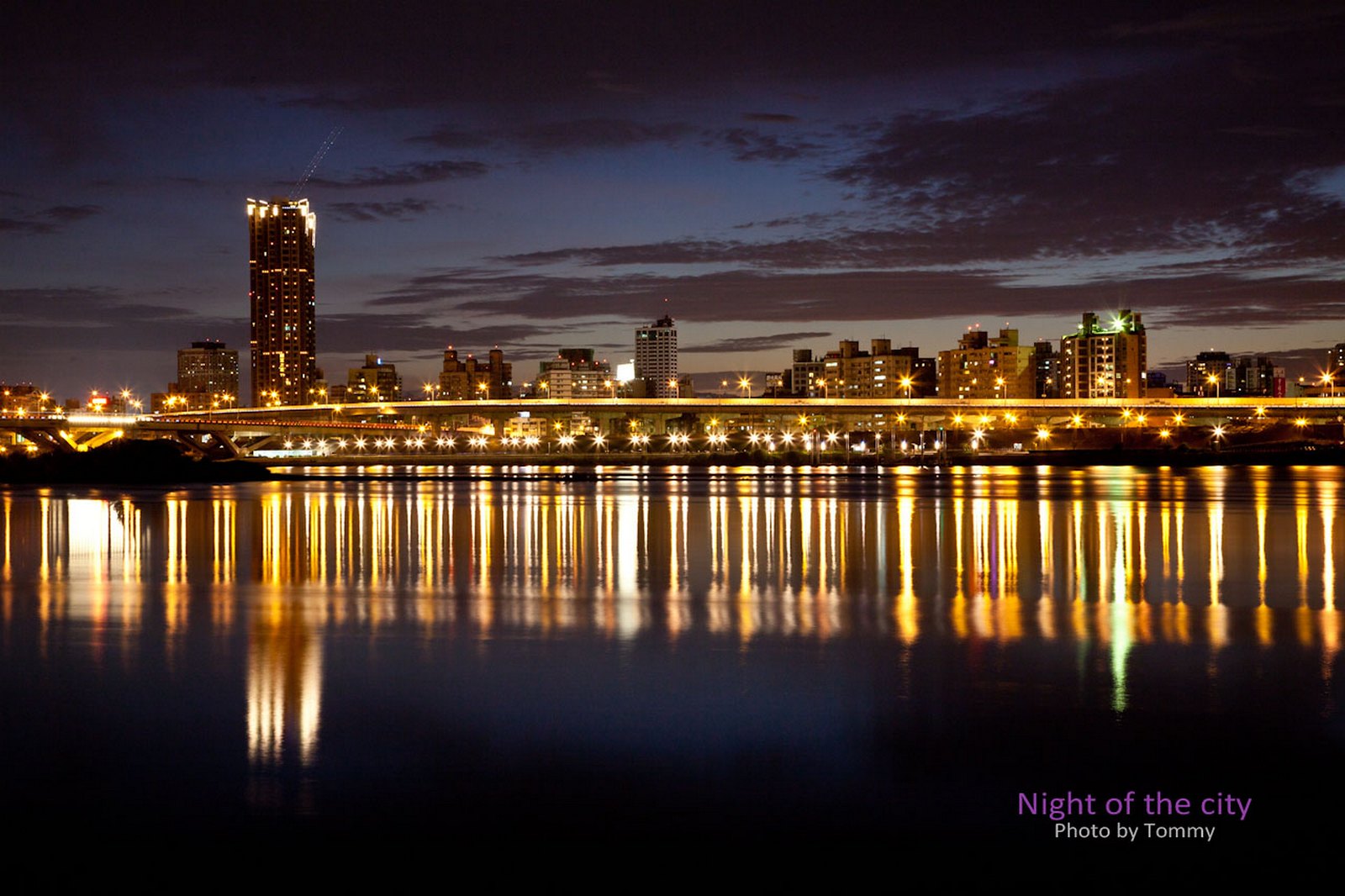This photograph, taken just after sunset, captures a mesmerizing night scene of a city skyline across a smooth, reflective body of water, possibly a river. The sky displays a gradient from a brownish hue near the horizon to deep blue and purple tones at the top, punctuated by dark clouds. The city's lights, predominantly golden yellow with hints of green, create a star-like effect, casting shimmering reflections on the water's surface. Prominent in the composition is a well-lit bridge that spans the image, while along the shoreline, numerous streetlights suggest pedestrian pathways. To the left, a significantly taller building, estimated at around 30 stories, stands out among other mid-rise structures, likely apartments and office buildings. The bottom right corner of the image features the caption "Night of the City," followed by "photo by Tommy" in white font, enhancing the photograph's atmospheric charm.